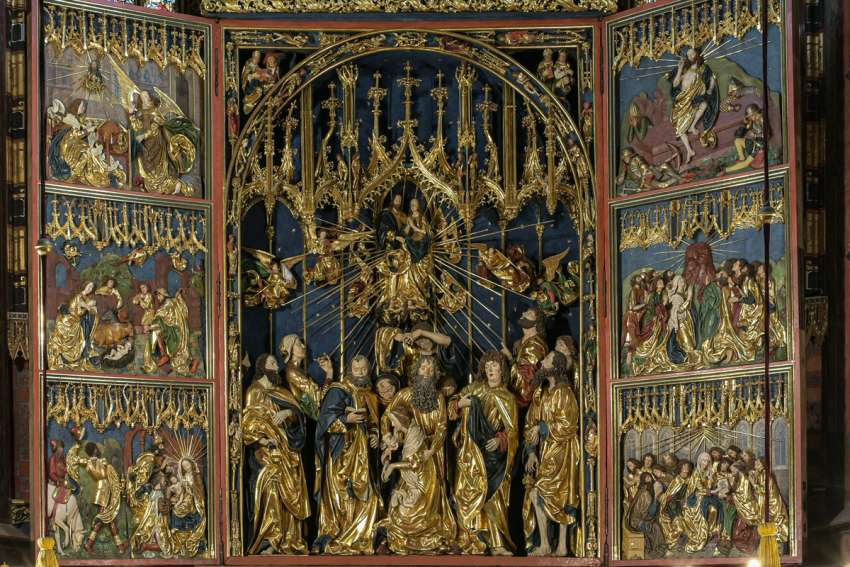The image is a detailed and ornate triptych, reminiscent of an altar piece commonly found in Catholic or Greek Orthodox churches, featuring a tri-fold presentation with an abundance of gold leaf and intricate designs. The central panel, arched at the top, prominently showcases a figure—likely Jesus—with his right hand raised, flanked by Mary and Joseph. Radiant beams extend outward from this trio. Below them, a scene including the apostles, distinguished by their gold-draped robes, beards, and staves, is depicted. The outer panels mirror each other with three stacked sections each. On the top of the left panel, angels are present with a star, possibly depicting the Nativity scene with Mary, Joseph, and baby Jesus. The middle section features another baby, an angel, and three other figures, while the bottom of the left panel shows Mary holding baby Jesus with the wise men approaching. The right panel’s top section depicts the Transfiguration, the middle tells a mountain-related story, and the bottom illustrates the Last Supper. The vibrant colors of gold, burgundy wood borders, deep blue backgrounds, and touches of reddish wine hues complement the figures adorned in gold and blue robes, each with halos signifying their holiness. The entire presentation, set within a church setting, is meticulously maintained and exudes a sense of sanctity and reverence.